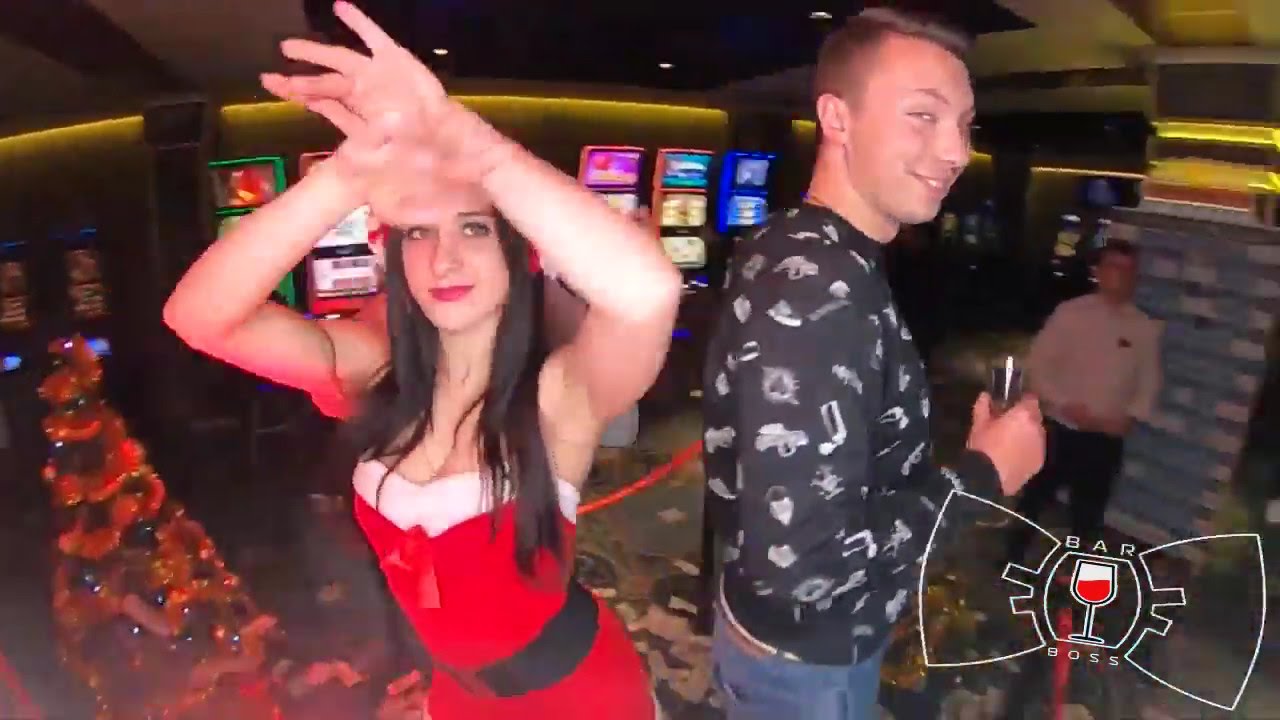The image captures a lively scene inside a bar with a festive, Christmas theme. At the center of the photograph are two main figures: a young woman on the left, wearing a distinctive Mrs. Santa Claus outfit. Her attire features a velvety red dress with a black belt, a puffy white top reminiscent of a Santa hat, and a red ribbon on the front. She appears to be in a joyous mood, with her arms raised as if she is dancing. To her right stands a man clad in blue jeans and a black shirt with a white design, holding a drink and directing a sly look towards the camera. The background reveals holiday cheer, with a Christmas tree adorned with decorations and the glow of neon lights. There are also slot machines and arcade games further highlighting the energetic atmosphere of the bar-casino hybrid setting. The image is marked with a "Bar Boss" logo in the lower right corner, indicative of the venue. In the far right periphery, there is a blurred figure dressed in a white shirt and black pants, adding to the crowded, festive ambiance.